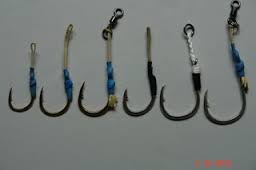This out-of-focus image showcases six fishing hooks of progressively increasing sizes, arranged from the smallest on the left to the largest on the right, set against a gray background. The hooks have sharp tips and metallic finishes, likely brass or another metal. Each hook features a small loop at the top for attaching a fishing line. Decorative colorful threads—in white, blue, and black—are tightly wrapped around the upper part of the hooks, possibly to distinguish between different styles or to add an aesthetic touch. A red date is present in the bottom right corner, though it remains too fuzzy to read.